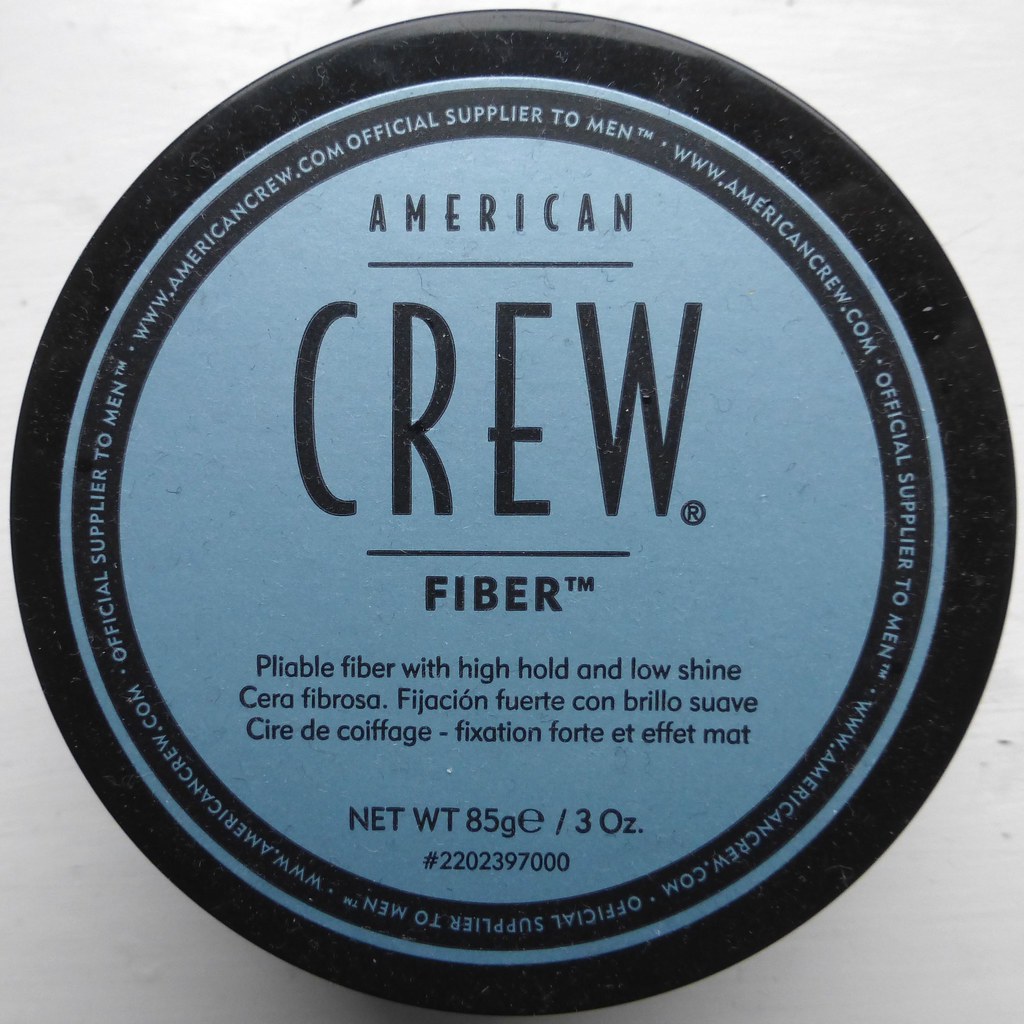This image features the circular top view of a container of American Crew Fiber hair product. Dominating the frame, the cap displays a light blue central label bordered by multiple black and gray rings. Surrounding the core is a black border inscribed repeatedly with "Official Supplier to Men" and "www.americancrew.com." The central part of the label features the brand name in a clear hierarchical arrangement: "American" in all caps at the top, followed by a line, then the word "CREW" in large all-caps with a registered trademark sign, and "FIBER" in large bold letters with a trademark symbol. Below this, the label reads "pliable fiber with high hold and low shine" along with its translations into multiple languages: "Cera Fibrosa," "Fixation fuerte con brillo suave," and "Cera de coifage - Fixation forte et effet mat." At the bottom, it specifies the net weight as "85 grams / 3 ounces," with the identification number "2202397000." The background of the image is a light gray, highlighting the product's prominent features.